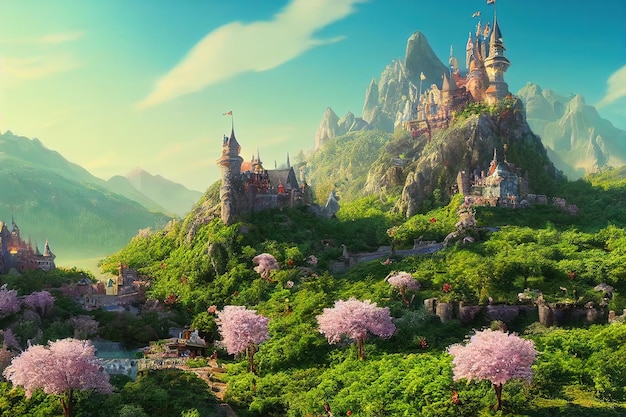The image appears to be a still from a computer-generated fantasy-themed video game, reminiscent of games like Myst. The scene features a series of majestic castles strategically perched on tall cliffs and mountain peaks. In the upper right-hand corner of the image, the largest castle dominates a sheer cliff, surrounded by imposing, jagged mountains that recede into the distance. Below this grand castle, a series of smaller castles and buildings nestle into the verdant valleys and hillsides, connected by bridges and paths winding through a lush landscape.

The foreground is rich with greenery, featuring trees, bushes, and low walls, contributing to the idyllic, magical setting. Among the greenery are taller, pink-flowering trees reminiscent of cherry blossoms, adding splashes of color to the predominantly green scenery. The landscape is bathed in a mix of crisp blue skies and fluffy white clouds, with hints of yellow sunlight fading in from the left, enhancing the whimsical and surreal atmosphere.

In summary, the scene is a vibrant tapestry of green, pink, blue, white, and gray, epitomizing a fantastical, fairytale landscape filled with exploration possibilities and a sense of awe-inspiring adventure.